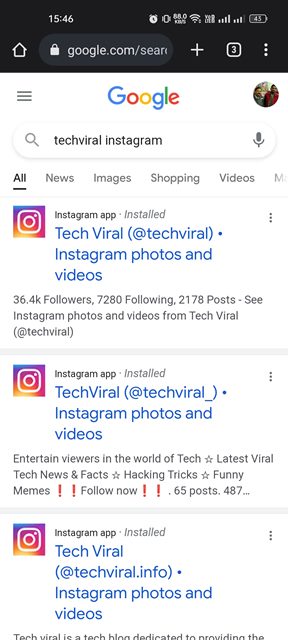This is a detailed screenshot from a tablet or smartphone displayed in military time, showing the current time as 15:46 in a black bezel. Various notifications populate the top bar: a clock icon, a vibrate mode indicator, an internet speed of 88.0 kb/s, a fully active Wi-Fi signal, and two cell phone signal bars indicating dual SIM usage. The battery icon shows 45%, signifying the remaining charge. 

In the navigation bar, a home icon is visible next to a URL with a lock symbol, displaying "google.com/search." To its right, there's a plus sign, a square with the number 3 inside a white border, and three vertical dots representing settings. 

Inside the white search area, the customary Google logo is displayed with the letters in their traditional colors: a blue 'G,' red 'O,' yellow 'O,' blue 'G,' green 'L,' and red 'E.' Adjacent to the logo is a profile picture depicting two individuals, one wearing a green shirt and the other a red shirt.

Below this, the search bar in an oval shape includes a gray magnifying glass icon and the text "TCHVIRAL," indicating a search for Technoviral on Instagram. To the right of the text, there is a gray microphone icon, part of an interface stylized like a pill with a 'C' beneath a line, possibly a clickable tab for categories. The categories include "All," which is bolded and underlined in black to show it is selected, and others like "News," "Images," "Shopping," "Videos," and another truncated to 'M.'

The main content area features various Instagram landing pages related to Technoviral Instagram, all hyperlinked in blue text, indicating clickable links. The background is white, and at the bottom, a partial description reads, "Technoviral is a tech blog dedicated to providing the..." with the remainder cut off.